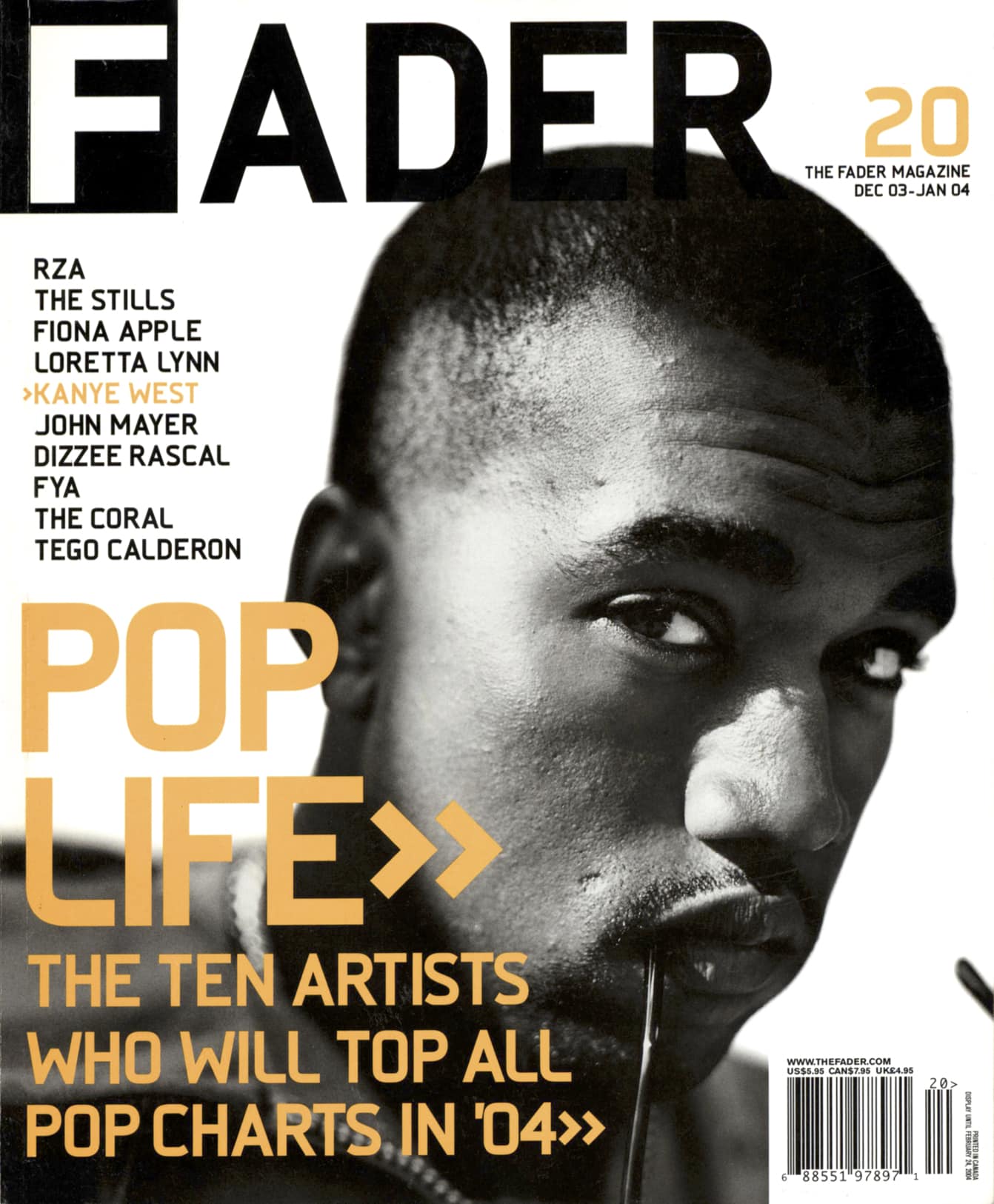This is the cover of Fader magazine, Issue 20, spanning December 3rd to January 4th. The background is completely white, and the magazine's title, "FADER," is displayed in black at the top. The cover features a black-and-white photograph of a young African-American man, presumably Kanye West, distinguished by his short haircut and straight-faced expression, with the earpieces of sunglasses in his mouth. Prominently, in yellow text, it says "Pop Life," highlighting the feature story about the ten artists who will top all pop charts in 2004. These ten artists are listed along the left side of the cover: RZA, The Stills, Fiona Apple, Loretta Lynn, John Mayer, Dizzee Rascal, FYA, The Coral, and Tego Calderon—all in black text except for Kanye West's name, which is highlighted in orange. The cover also includes a scan code at the bottom right corner.